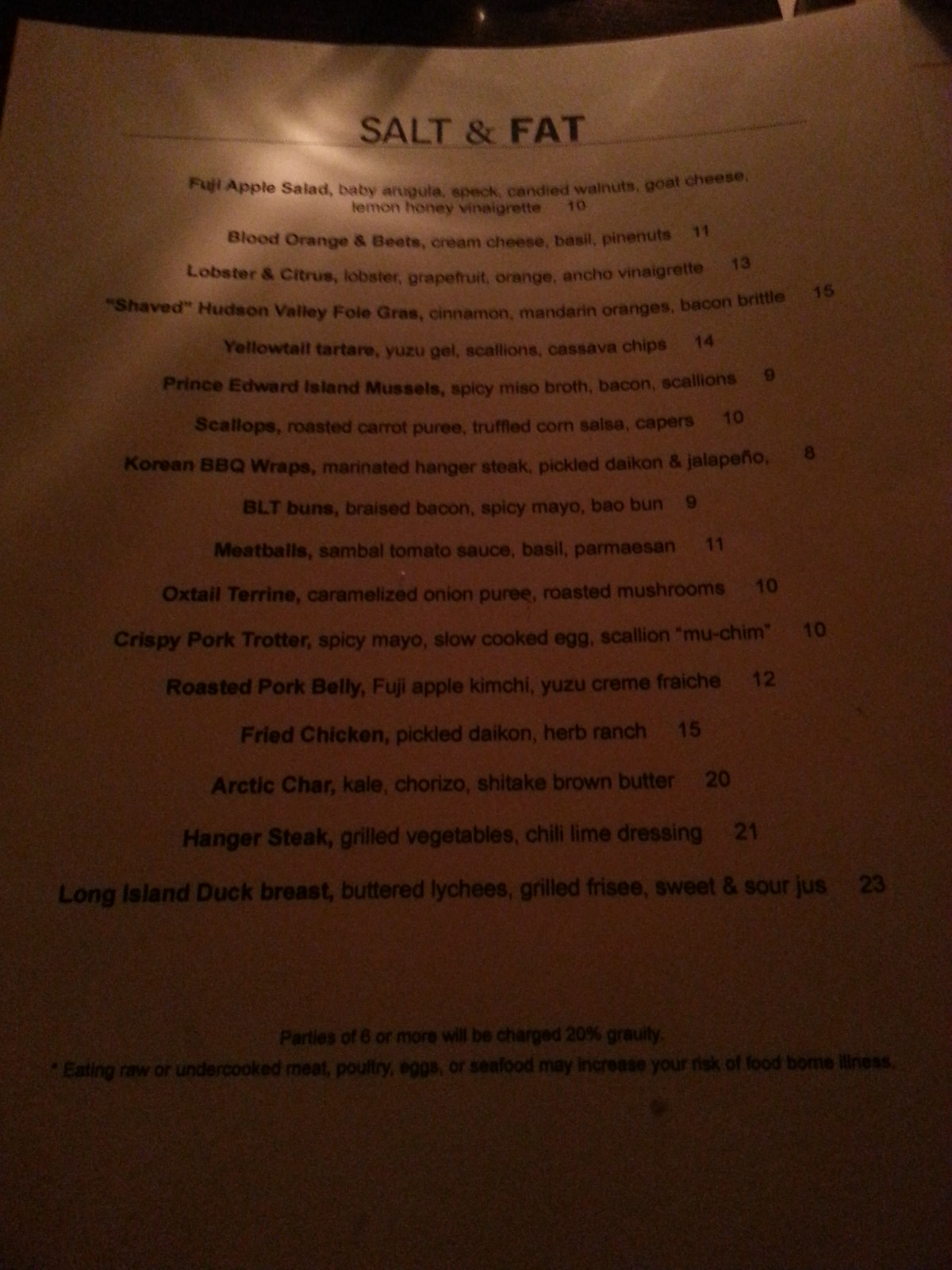The image is a dimly lit, color photograph of a portrait-oriented menu from a restaurant called Salt and Fat. The menu, printed on a tan or white background, is primarily in shadow, with a small amount of light illuminating the center top, creating a challenge in reading the text, especially towards the bottom. The headline at the top of the page prominently reads "SALT and FAT" in all caps, underscored by a line. Below this are various menu items, each accompanied by pricing information. The entrees listed include Fuji Apple Salad, Blood Orange and Beets, Lobster and Citrus, Shaved Hudson Valley Foie Gras, Yellowtail Tartare, Prince Edward Island Mussels, Scallops, Korean Barbecue Wings, BLT Buns, Meatballs, Oxtail Terrine, Crispy Pork Trotter, Roasted Pork Belly, Fried Chicken, Arctic Char, Hanger Steak, and Long Island Duck Breast with Butter Lychee and Grilled Frosé Sweet and Sour Jus for $29. Towards the bottom, the text becomes increasingly illegible due to the shadows. The menu is described in a style of Photographic Realism Representationalism.